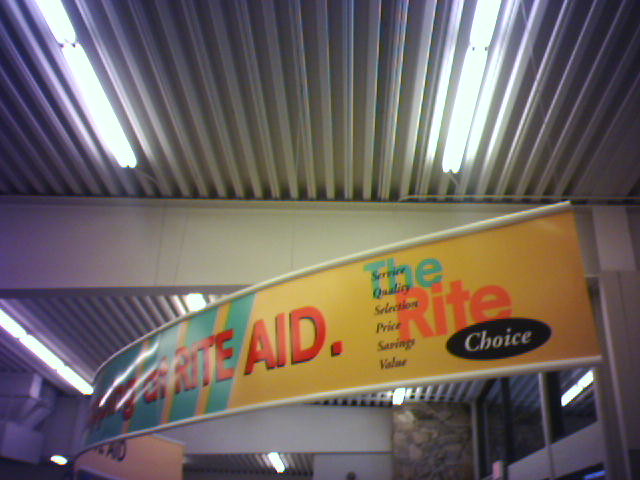The photograph captures the interior of a Rite Aid store. Central to the image is a curved, yellow sign in the foreground, prominently displaying the phrase "The Right Choice." The words are color-coded: "The" in light blue, "Right" in orange, and "Choice" in a round, black bubble with white lettering. From the top of the sign, arranged vertically down the right side, are the words "Service," "Quality," "Selection," "Price," "Savings," and "Value" in descending order. Surrounding the sign are diagonal turquoise stripes starting from the "E" in "Right". 

To the right of the sign is the continuation of the store name "Rite Aid" on the curve, wrapping around the display. Above, the ceiling is made of corrugated steel with a central beam also constructed from steel, providing structural support. On this ceiling are two groups of lighting: the first group consists of two fluorescent lights, while the second group, slightly more distant, includes three lights, though only the rightmost light is fully visible. Behind this section, there is a wall with an additional fluorescent light glowing in the background.